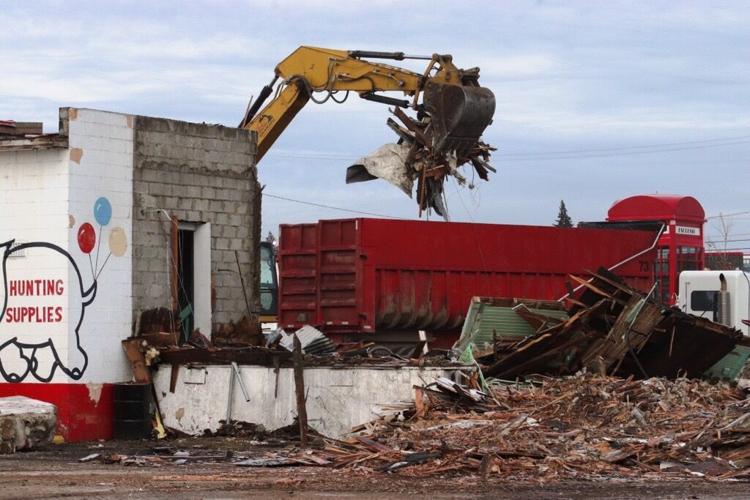The photo, taken outdoors on a partly cloudy day under a vibrant blue sky, features a chaotic scene of demolition and cleanup. Dominating the background is a yellow crane or backhoe lifting various debris and rubble. On the far left is a partially destroyed white-painted building, bearing a red-outlined elephant with the phrase "Hunting Supplies" inside. The building's backside, adorned with the elephant's tail and three balloons, adds a whimsical touch amidst the destruction. Scattered around the ground are numerous 2x4s and miscellaneous trash, creating a disordered industrial atmosphere. To the right, a classic red British telephone booth stands beside several red dumpsters filled with debris being loaded by the machinery. Above it all, power lines stretch across the sky, and a white tractor trailer with a visible exhaust and smokestack is parked in the background. The scene captures the stark contrast between the ongoing demolition and the remnants of the building's former purpose.